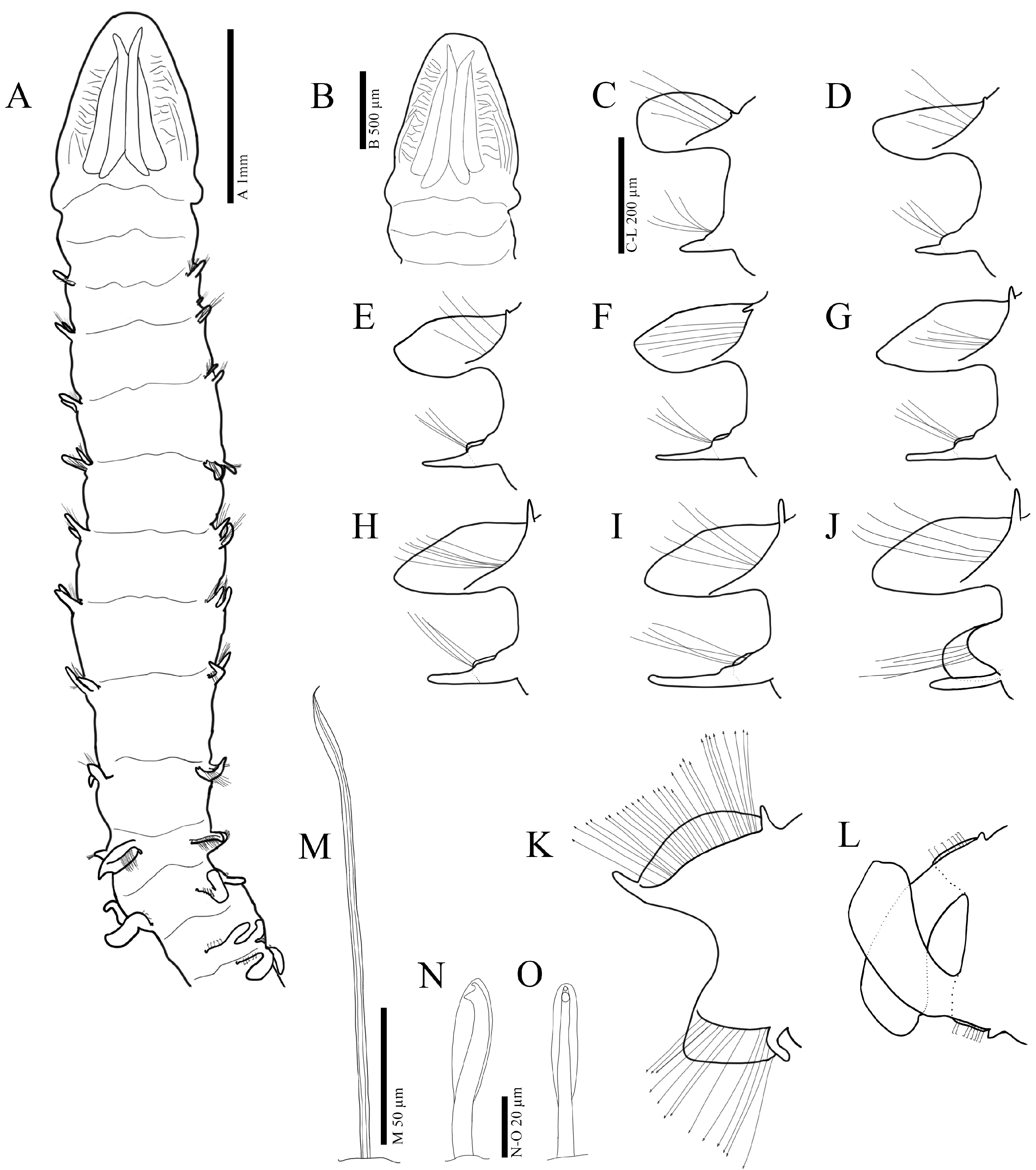This detailed illustration appears to depict a microscopic, worm-like animal, potentially a centipede, shown from various angles and magnifications. The primary diagram (A) displays the full body of the creature, including a head measuring approximately one millimeter. Other diagrams (B through O) break down specific parts of the organism: B focuses on the head with a measurement of 500 micrometers, and C further narrows down to a 200-micrometer section. Each segment is meticulously annotated with measurements, showing different appendages and body parts. Diagrams D through J showcase individual limbs with hair-like structures extending outward. Sections K and L highlight parts of the torso and arm regions. Finally, sections M, N, and O detail slender, stem-like structures with lengths of 50 micrometers down to 20 micrometers, possibly corresponding to either a tail or specialized feeding apparatus. The diagram is rendered in black ink on a white background, suggestive of an older illustration style, possibly from the mid-20th century.